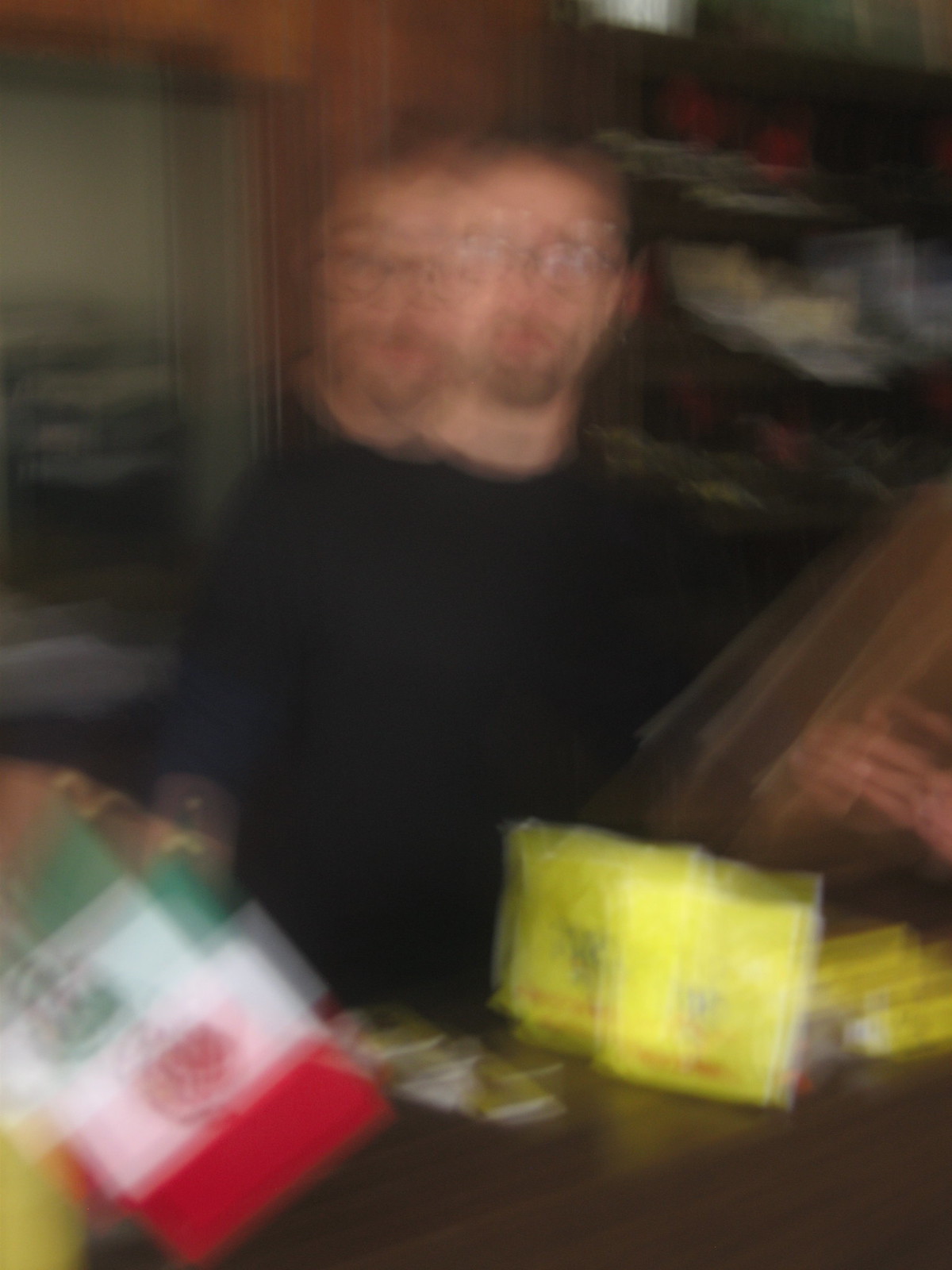In this extremely blurry photograph, there is a man whose image is distorted, making it appear as though he has double heads. He is wearing glasses and has some facial hair. He is dressed in a dark-colored shirt. There is a dark wood-colored table in front of him. The background features what seems to be orangey-toned wood. A Mexican flag with green, white, and red stripes is visible, adding a splash of color to the scene. On the table, there is some yellow packaging. The man is holding an indistinguishable, super blurry object that looks like an orangey-brown blob.